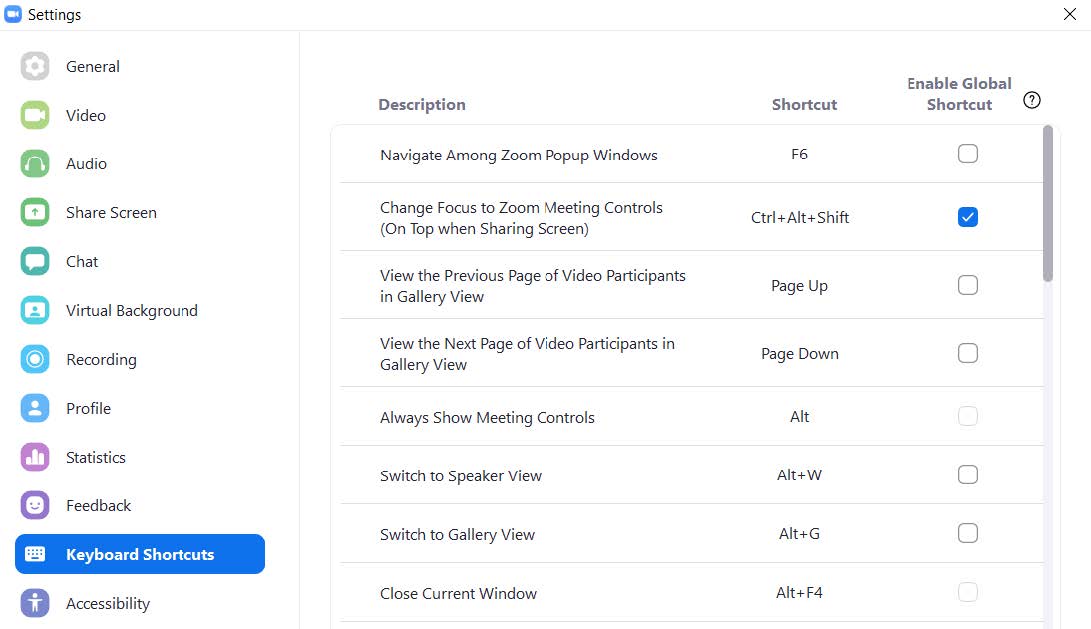This image is a screenshot of a Zoom application settings menu displayed on a laptop screen. The interface is characterized by a white background with black text and an assortment of colorful icons alongside each menu item. At the top of the screen, the word "Settings" is prominently displayed, accompanied by the Zoom icon, signifying that these settings pertain to the Zoom application.

On the left side of the screen, there is a vertical menu that categorizes various settings options. Each category is identified by both text and corresponding icons: 
- "General" with a gear icon,
- "Video" with a camera icon,
- "Audio" with headphones, 
- "Share Screen," 
- "Chat," 
- "Virtual Background," 
- "Recording," 
- "Profile," 
- "Statistics," 
- "Feedback," 
- "Keyboard Shortcuts," 
- "Accessibility."

The highlighted item in this menu is "Keyboard Shortcuts," indicated by a blue bar. Selecting this has opened a detailed sub-menu on the right side of the screen, showcasing various keyboard shortcut options. At the top of this section, there is an option to "Enable Global Shortcut" followed by a list of specific shortcuts.

The first listed shortcut is "Navigate among Zoom pop-up windows," associated with the F6 key. Directly below this, a checked option reads "Change focus to Zoom meeting controls," among other items. Each shortcut description is given a checkbox to indicate whether it is enabled or not.